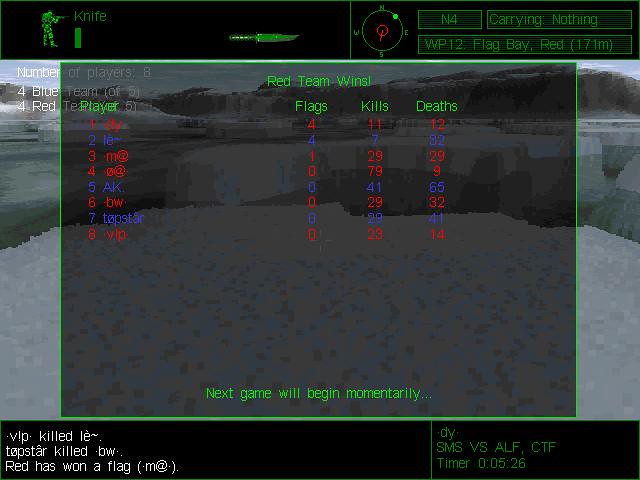The image is a horizontally rectangular screen grab from a video game, bordered by horizontal black banners at the top and bottom. On the top banner, to the left, there's an image of a player in the game accompanied by the word "Knife" in neon green text. On the upper right of the same banner, there are three horizontally rectangular boxes displaying various game-related information.

The game’s background features an expanse of large ice pieces with water in between them. Overlaying this scene is a semi-transparent gray box. Within this box, it states "Red Team Wins" in prominent text, followed by four columns labeled "Player," "Flags," "Kills," and "Deaths," each listing corresponding information.

At the bottom of this gray box, a message reads: "Next game will begin momentarily."